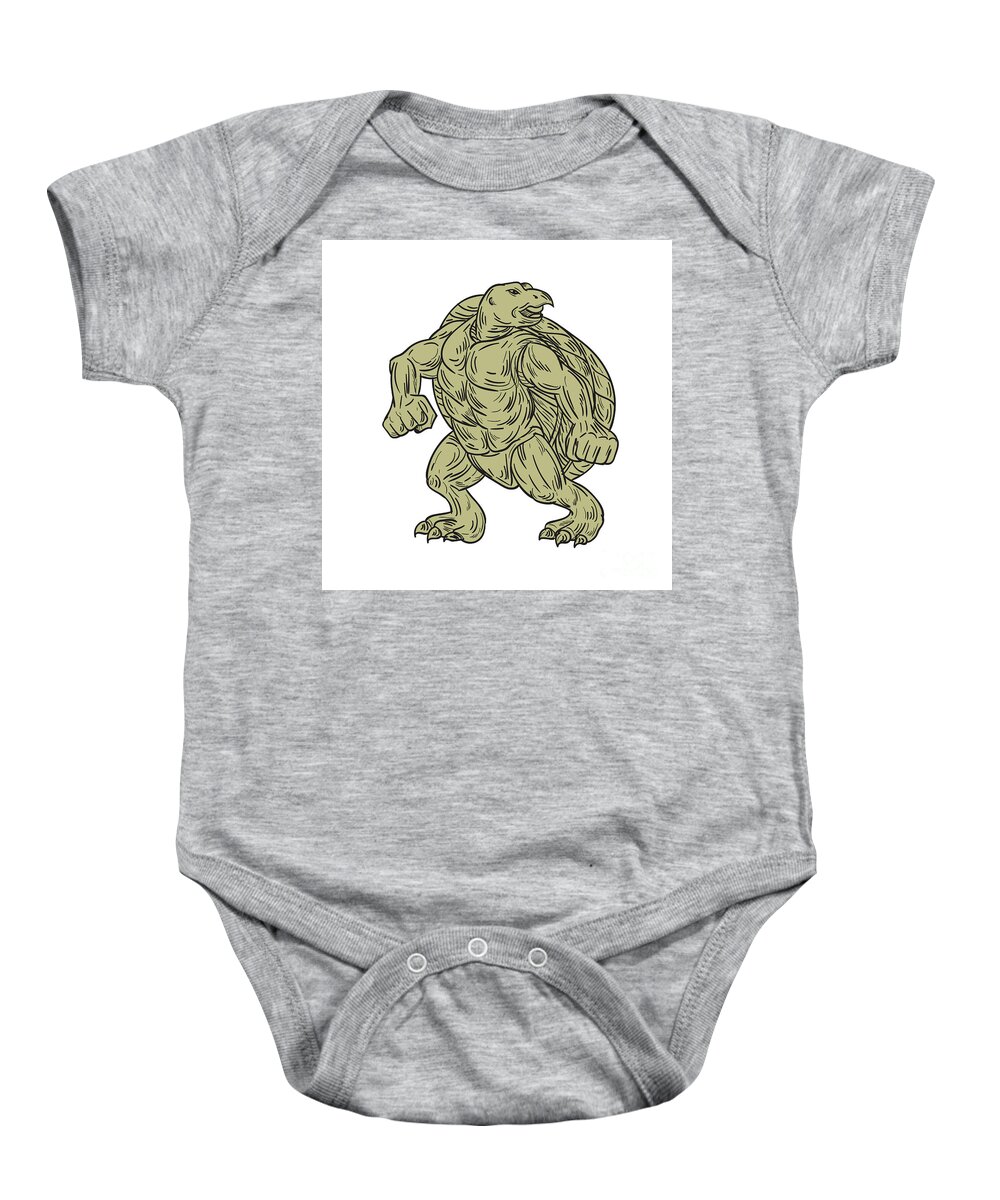The image depicts a short-sleeved, dark gray baby onesie facing the camera, with the bottom featuring a flap that snaps with three white buttons for easy diaper changes. At the top center of the onesie, there is a white rectangular box displaying a detailed, cartoon-like graphic of a green turtle. The turtle stands upright with a muscular build, similar to a character from a traditional cartoon or a ninja turtle. Its chest faces forward while it clenches its fists, preparing for action. Its feet point slightly to the left, and its head is turned to the right. The design is simplistic yet striking, with no additional embellishments on the rest of the onesie.